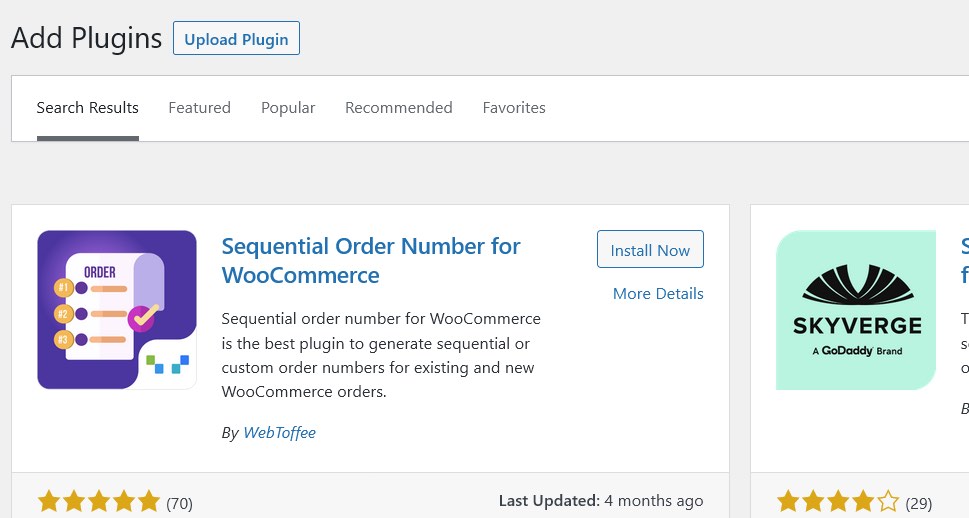**Caption:**

This image depicts a webpage dedicated to advertising various plugins. The page is structured with a gray background and predominantly black and white color scheme, featuring distinct sections such as “Search Results,” “Featured,” “Popular,” “Recommended,” and “Favorites” across the top bar. At the top, a prominent title reads "Add Plugins," accompanied by a small blue link allowing users to upload their own plugins.

Central on the page is the "Sequential Order Number for WooCommerce" plugin by Web Toffee. This plugin is highlighted with the option to "Install Now" or access "More Details." It boasts a stellar five-star rating from 70 reviews and was last updated four months ago. This plugin's icon is set against a purple background, depicting a stylized receipt.

To the right, there's an ad for another plugin, "SkyVerge, a GoDaddy brand," displaying an average rating of four stars from 29 reviews. The SkyVerge plugin has a very light green icon with black text, although the full details of the ad are partially cut off in the image. The page layout includes several square boxes in white, creating a clean and organized appearance.